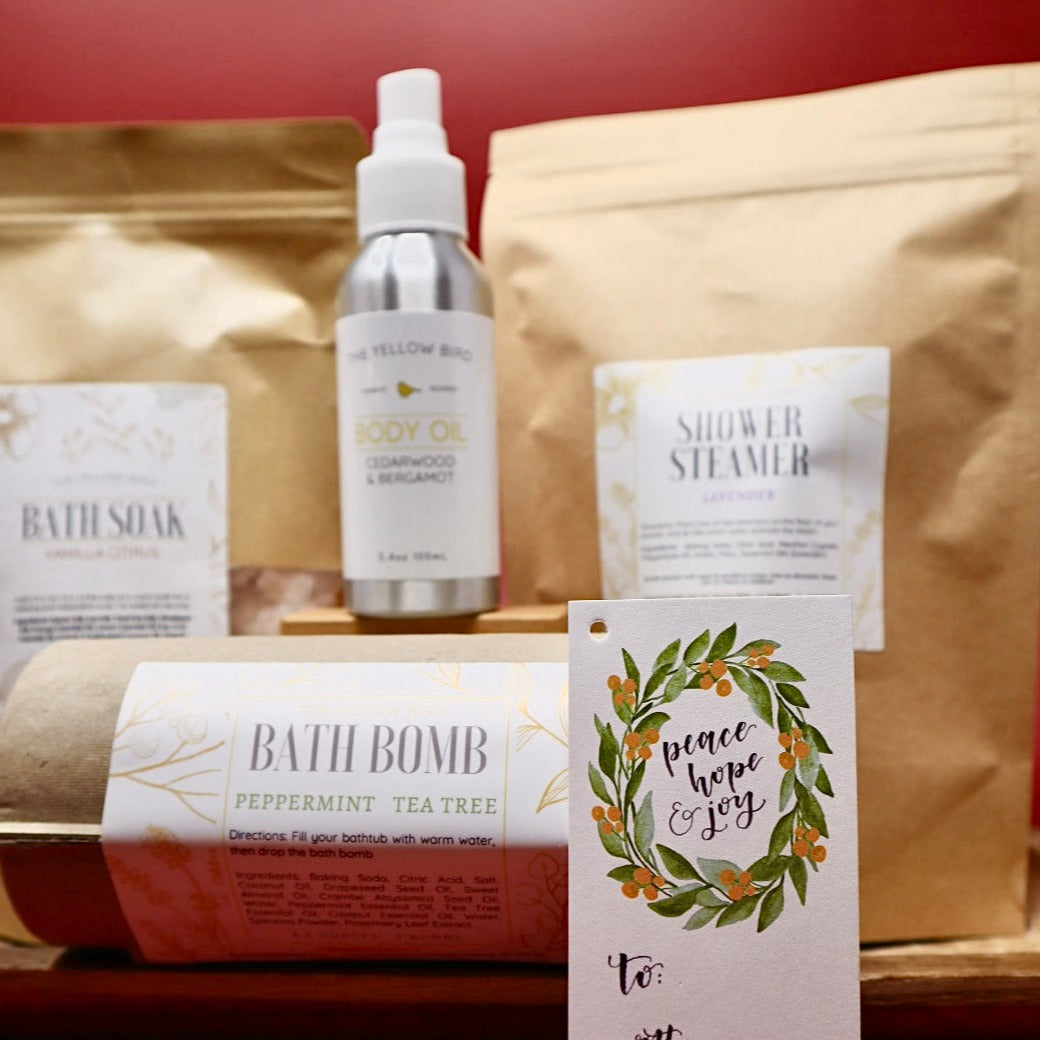A close-up, square-shaped photograph showcases a charming, homemade spa treatment kit designed for self-care. The kit includes four products: a bath soak, a shower steamer, a bath bomb, and a body oil. The bath soak and shower steamer are packaged in large, brown paper bags with white labels adorned with gold designs and black text. The bath soak label appears on the left, while the shower steamer is on the right. Positioned centrally, a silver spray canister labeled "Body Oil" in yellow text with "Cedar Wood and Bergamot" in black rests on a small, barely visible wooden block. Below the canister, a cylindrical cardboard tube labeled "Bath Bomb" with intricate gold tree branches and black text details its Peppermint Tea Tree fragrance, along with usage instructions. In the foreground, a white gift card with a hole punch in the upper left corner features a green wreath with orange berries and the cursive message "Peace, Hope, and Joy." Beneath the message are "To" and "From" fields for personal gifting. The backdrop includes a dark red wall, adding contrast to the predominantly white and brown color palette of the kit.